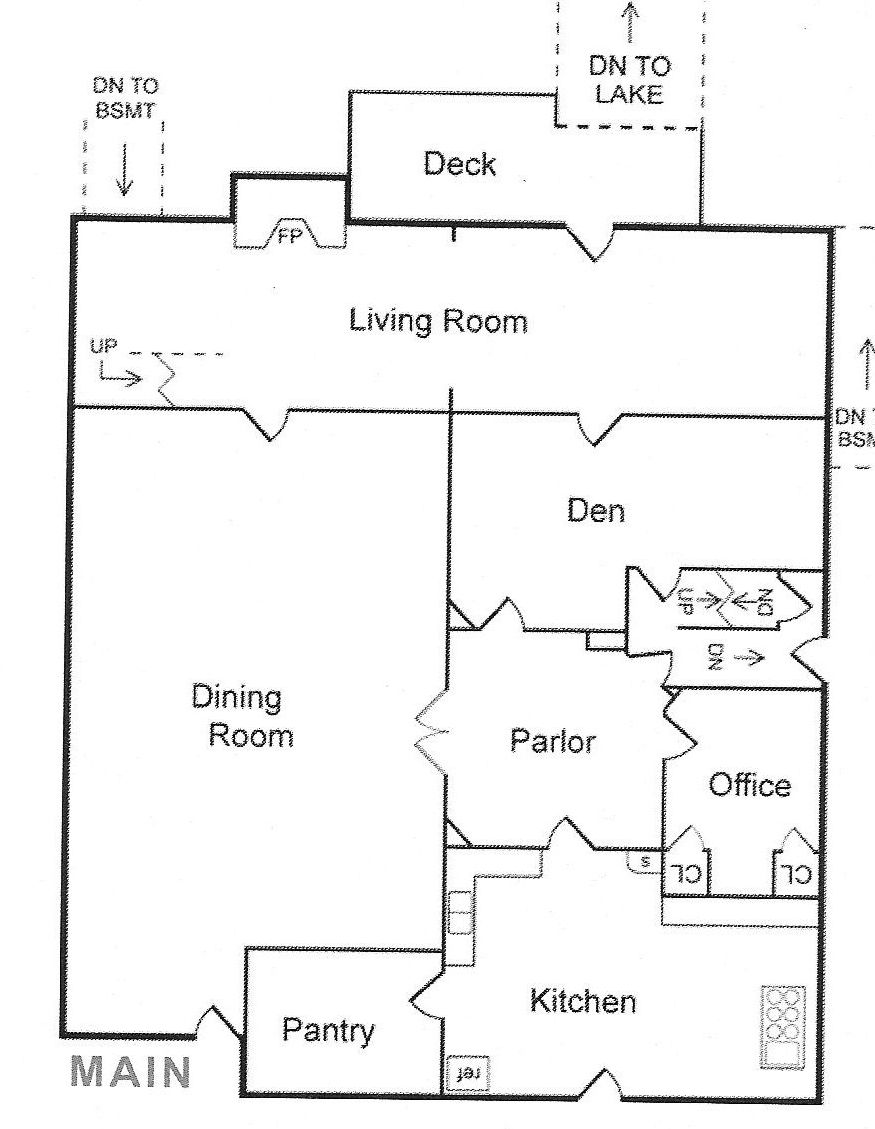This image is a black and white architectural drawing of a house, viewed from above. The house is divided into various labeled sections, each depicting different parts of the home.

In the upper left corner, a dotted line corridor labeled "DN to BSMT" with an arrow pointing downward indicates the way to the basement. To the top of the structure, there's a depicted deck. An additional dotted column with an arrow labeled "DN to lake" suggests a pathway leading down to a lake.

The upper portion of the house is designated as the living room, which takes up just under a third of this section. The boundaries of the living room are marked by lines, with two doors positioned on the lower right and lower left corners. Below and to the left of the living room lies the dining room, which extends to the very bottom of this area. In the lower right corner of the dining room is a section marked as the pantry. The main entrance door is located at the bottom left of the dining room.

To the right of the living room, the drawing features a den, beneath which is a parlor at the center of the home, and to the bottom right, a kitchen. There are detailed door drawings indicating the entry and exit points for each room. To the right of the parlor, there's an office, with clearly depicted open doors signaling access to the different areas. Additionally, to the right of the den, upstairs and downstairs staircases are indicated, providing internal connectivity throughout the house.